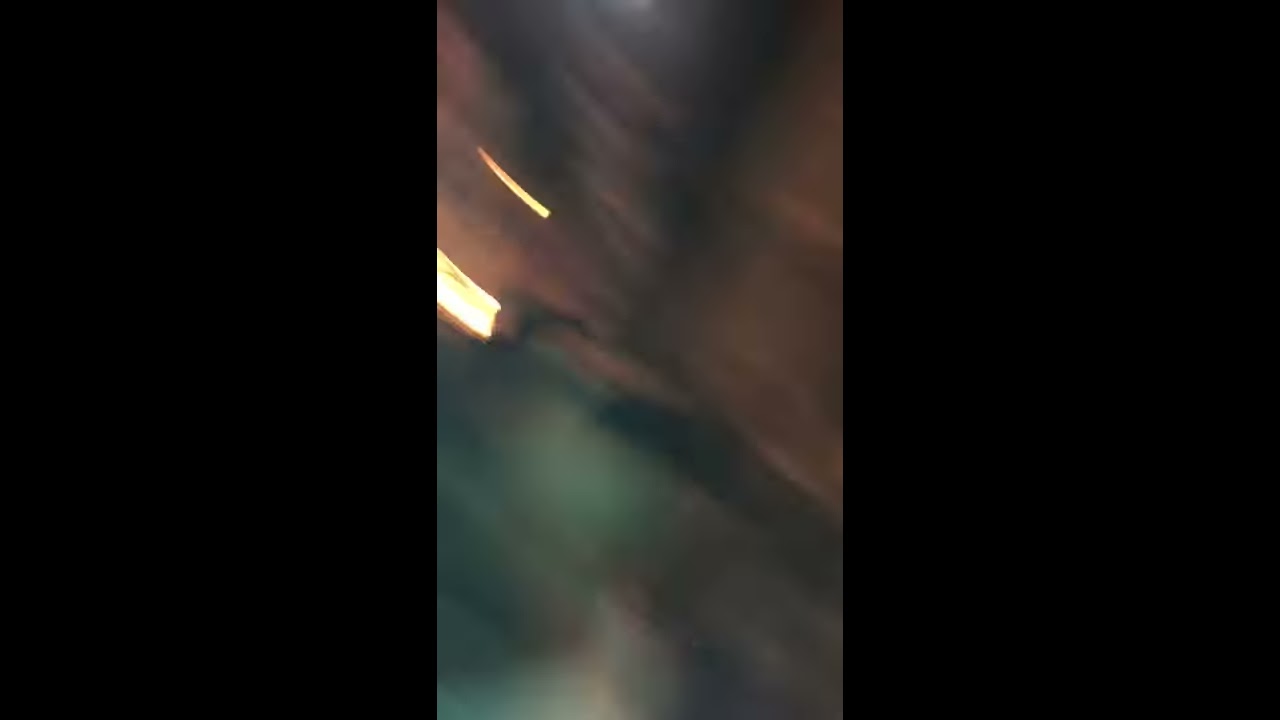The image is almost completely indistinguishable due to significant blurriness. It was taken vertically, making it taller than it is wide, and most of the photograph is dominated by thick black rectangles on the far left and right sides. The center portion of the image is an unfocused blur of colors. Dominant hues include greens, reds, browns, grays, blacks, and slight hints of white. A distinguishable feature within the blur is the presence of two bright yellow lights, which appear as long rectangular streaks positioned in the middle left area. The upper part of the blurred area has more reddish, brownish tones, while the lower part shows greens, blacks, and some grays. The photo appears to have been taken indoors, possibly with a phone, and was captured in motion, making it difficult to identify any clear outlines or definitive objects. Overall, the image lacks any text and is primarily a smudge of colors and shapes.